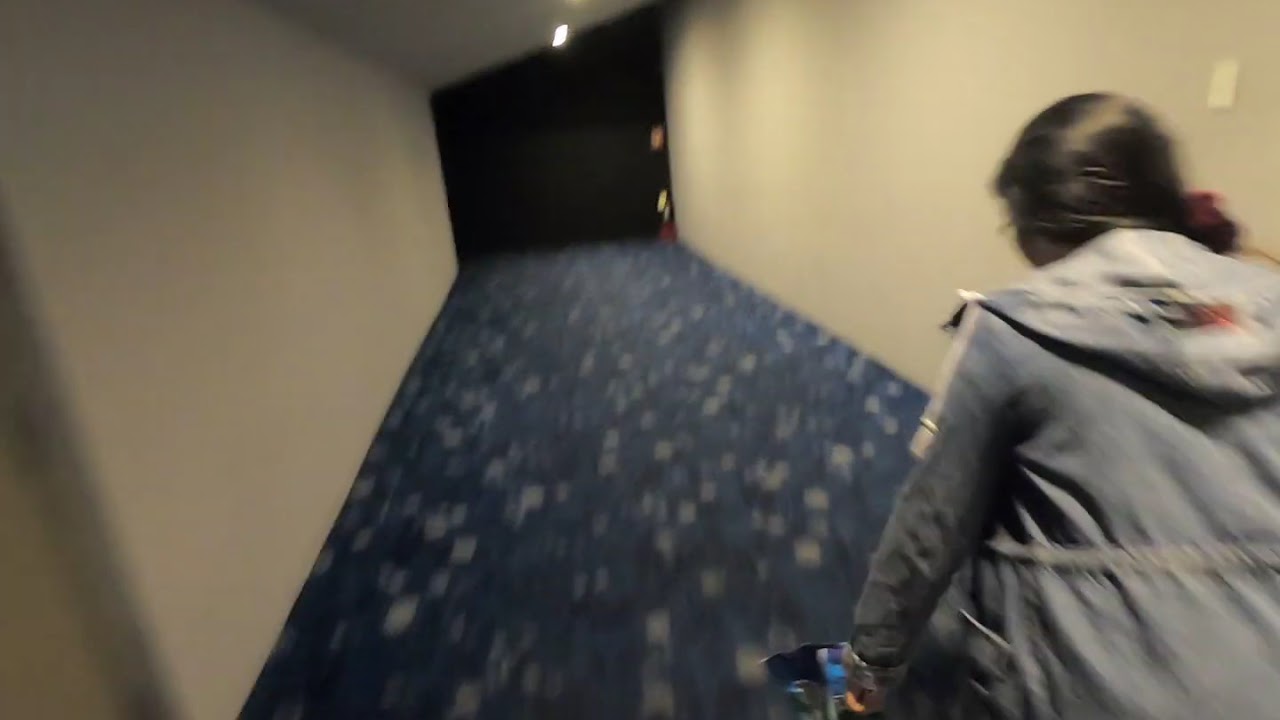The image depicts a blurry but detailed scene of a woman walking quickly or running down what appears to be a carpeted hallway, possibly in an apartment building or hotel. The carpet is navy blue with white speckles, evoking the aesthetic of a movie theater walkway. The walls on either side are white, and there is a door on the left side of the hallway, adding to the residential or hospitality feel. The ceiling in the foreground is slanted, leading to a dark, almost black void at the far end of the hallway, which is illuminated by a bright light overhead. The woman has dark hair pulled back into a ponytail with a maroon scrunchie and is dressed in a gray hoodie. She appears to be holding or pushing something - potentially cleaning equipment or a cart - though the blur of the photograph obscures these details. Despite the motion blur, the impression is of a scene filled with movement, defined by a speckled carpet and stark lighting contrasts.